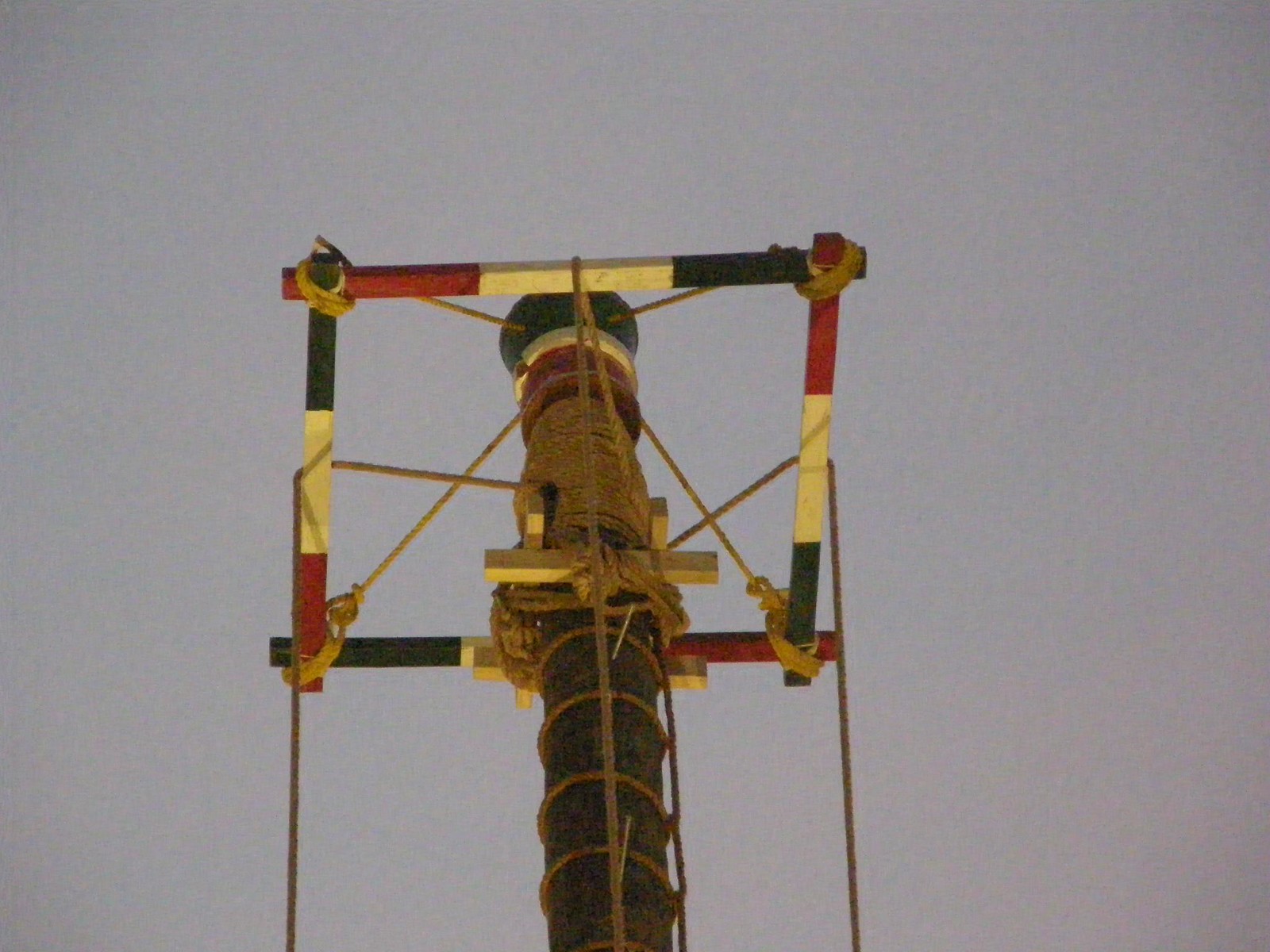The color photograph captures a tall, slender pole resembling a thick tree trunk, soaring upward against an overcast gray sky. The focal point at the top of this pole is a handcrafted square frame constructed from four wooden beams, each corner meticulously tied with yellow rope. This frame, adorned in the vibrant colors of red, yellow, and black, serves as the base from which more ropes descend, wrapping around the pole. This structure appears familiar as it closely resembles the traditional setup used by renowned acrobatic indigenous performance artists from Mexico, noted for their spectacular aerial feats during festivals. Although the performers are not visible in this shot, the iconic red, white, and green colors hint at the cultural significance and festive purpose of this framework. The image is detailed and clear, emphasizing the craftsmanship and cultural context of this intriguing structure.